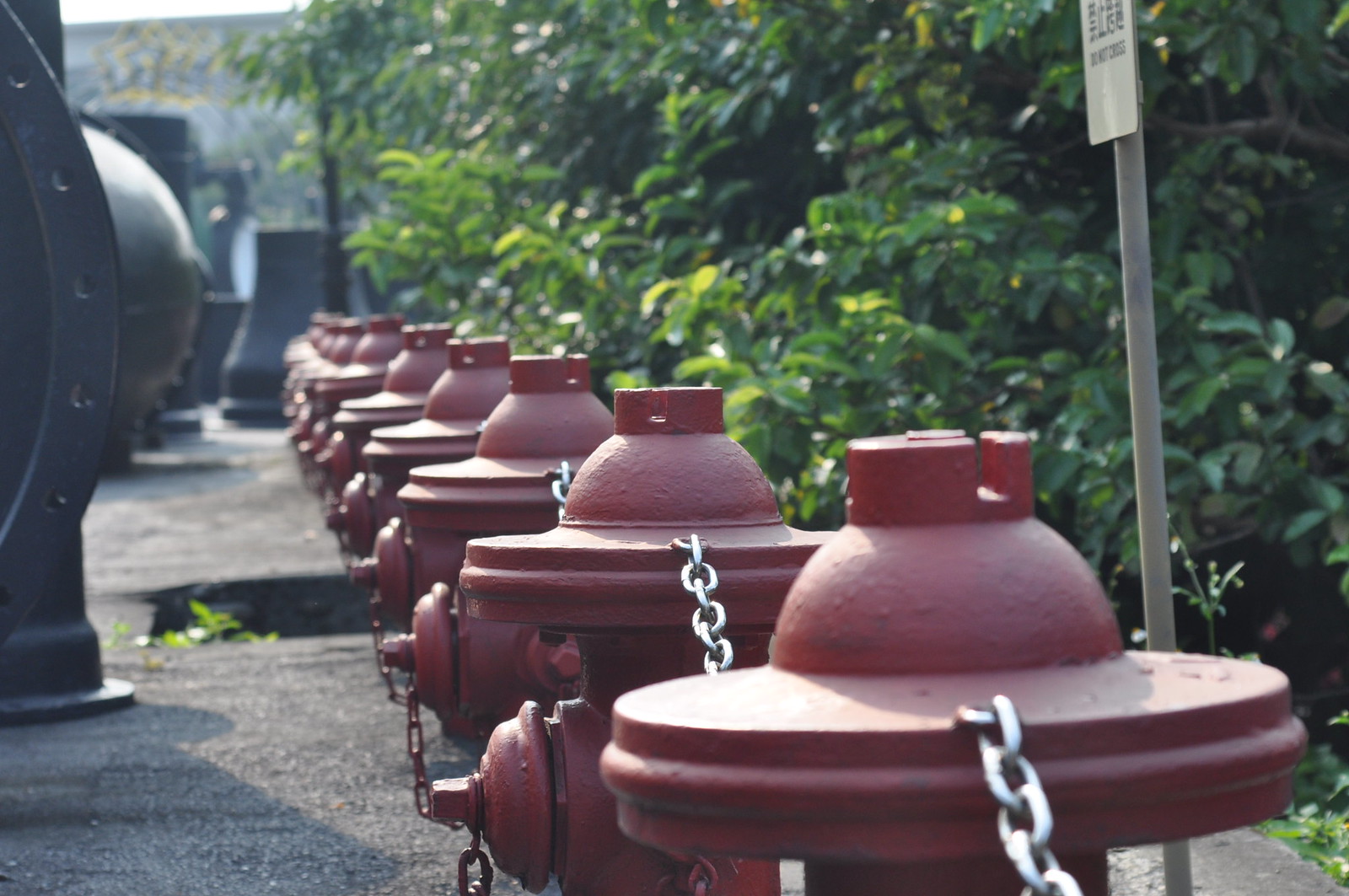This digital photograph captures a line of approximately twelve medium-sized red fire hydrants, chained together and mounted on a pavement that runs from the bottom right to the top left of the image. The hydrants gradually recede into the distance, creating a linear perspective. Behind the hydrants, there is a backdrop of dense green shrubbery and small trees with abundant green leaves. A sign near the back right side of the hydrants is partially visible but mostly unreadable, with some indication that it includes a message about not crossing. On the left-hand side of the image, an off-colored red brick wall or building is partially visible, along with a substantial black metal pipe extending towards the rear. Scattered gaps in the pavement add texture to the ground, and some vaguely defined metal structures, possibly circular vents or other industrial objects, are also present. The concrete walkway and the presence of a distant building or structure round out the scene, providing a sense of an organized yet slightly worn setting.